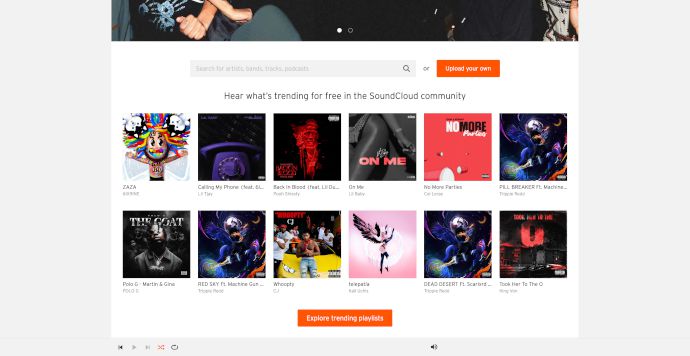Screenshot of the SoundCloud Website Displaying Trending Tracks

The screenshot captures a dynamic section of the SoundCloud website, specifically the trending tracks page. At the top of the page, there is a partially visible image of a crowd at an event or concert, suggesting a lively and musical atmosphere. Below this header, a search bar takes center stage with the placeholder text, "Search for artists, bands, tracks, podcasts," accompanied by an orange button labeled "Upload your own."

The primary focus of the page is the "Hear What's Trending for Free in the SoundCloud Community" section. This area showcases a grid layout filled with various album covers or track thumbnails, each providing details such as the track title and the artist's name. Amongst the highlighted SoundCloud artists and their tracks are:

- "ZAZA" by 6ix9ine
- "Calling My Phone" by Lil Tjay
- "Back in Blood" featuring Lil Durk by Pooh Shiesty
- "On Me" by Lil Baby
- "No More Parties" by Coi Leray
- "Pill Breaker" by Trippie Redd featuring Machine Gun Kelly and blackbear
- "GOAT" by Polo G
- "RED SKY" by Machine Gun Kelly
- "Whoopty" by CJ
- "Intergalactic" by Kid Cudi
- "Dead Desert" by Scarlxrd
- "Took Her to the O" by King Von

At the bottom of the page, icon buttons for playback controls, volume adjustment, and other interactive features are visible, suggesting an integrated, user-friendly audio player. The website showcases an array of diverse and emerging artists, many of whom have gone on to achieve greater fame. Despite the variety of talent, the user expresses a critical opinion on the quality of the music, describing it as "garbage."